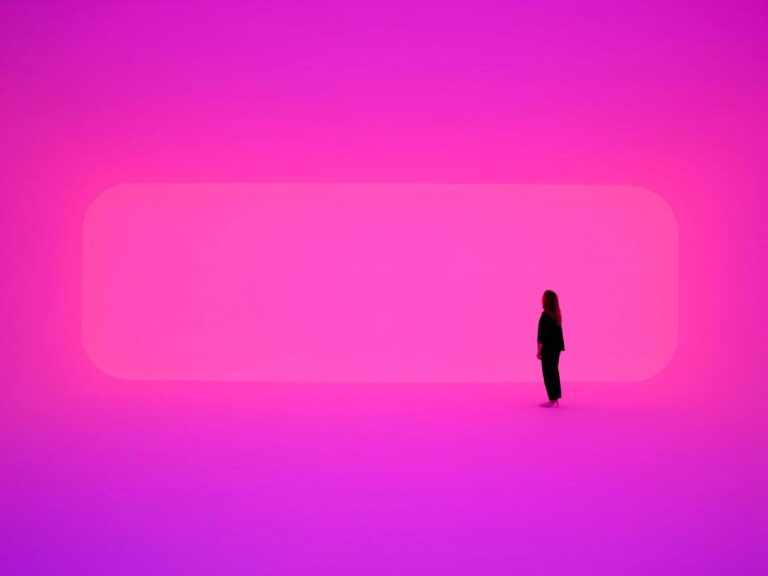The image features a woman standing against a vibrant background that transitions from a deep purple at the corners to a vivid bright pink at the center. Overlaid in the central area is a rounded-edged rectangle in a slightly darker shade of pink than the surrounding area. The foreground showcases a woman positioned to the right of this rounded rectangle, standing in profile and turned slightly towards it. She is dressed in dark attire, consisting of a jacket that ends just below her elbows and pants that stop above her ankles, leaving her hands and feet exposed. Her long brown hair cascades past her shoulders, and her skin, affected by the pink hue of the background, appears slightly pinkish. She gazes diagonally upward at the rectangle, creating a curious interaction between herself and the geometric shape behind her.